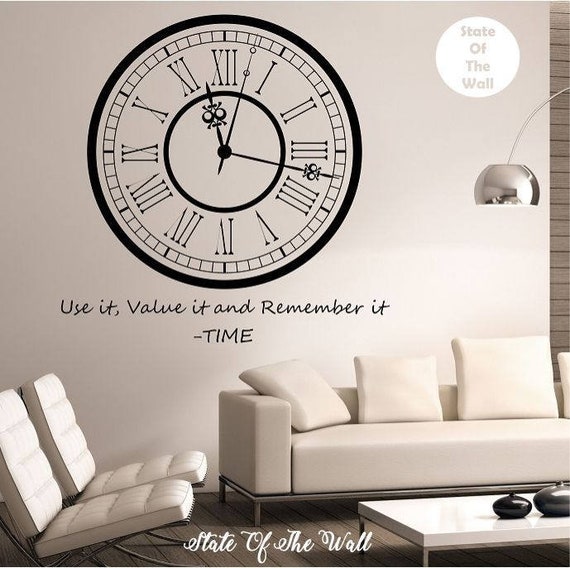The photograph captures a modern, minimalist room with a white couch adorned with white pillows. To the left of the couch, there are two chairs with white cushions, all featuring chrome metal bases at the bottom. The backdrop includes a white wall that prominently displays an old-style analog clock with Roman numerals. The clock shows the hour hand between 11 and 12, the minute hand between the 3 and 4, and the second hand between the 12 and 1. Below the clock is a cursive quote that reads, "Use it, value it, and remember it. Time." The bottom of the wall features another cursive inscription in white that states, "State of the Wall." Additionally, at the top right corner of the wall, there is a white circle containing the same phrase, "State of the Wall," written inside.